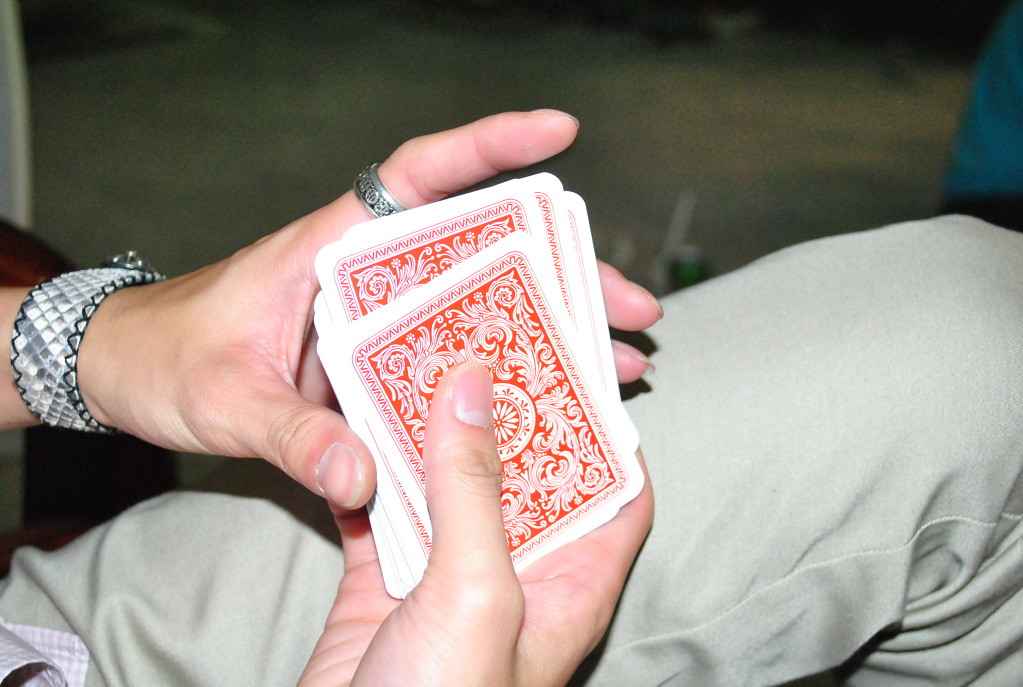The image is a close-up photograph of a woman's hands. On her left hand, she wears a wide, flat bracelet made of gray and white woven beads, complemented by black stitching along the edges. Her wrist looks delicate. She is also wearing a silver band ring with intricate Celtic designs on her forefinger.

Both of her hands are holding a deck of playing cards, which have a white background and a red design. The woman is dressed in pale gray or off-white chinos, possibly in a natural color shade. Only her left leg up to the knee, which is bent, is visible in the picture, indicating she is sitting on a chair or couch.

The background reveals a medium brown floor with darker shaded areas, giving a glimpse of the room's setting.